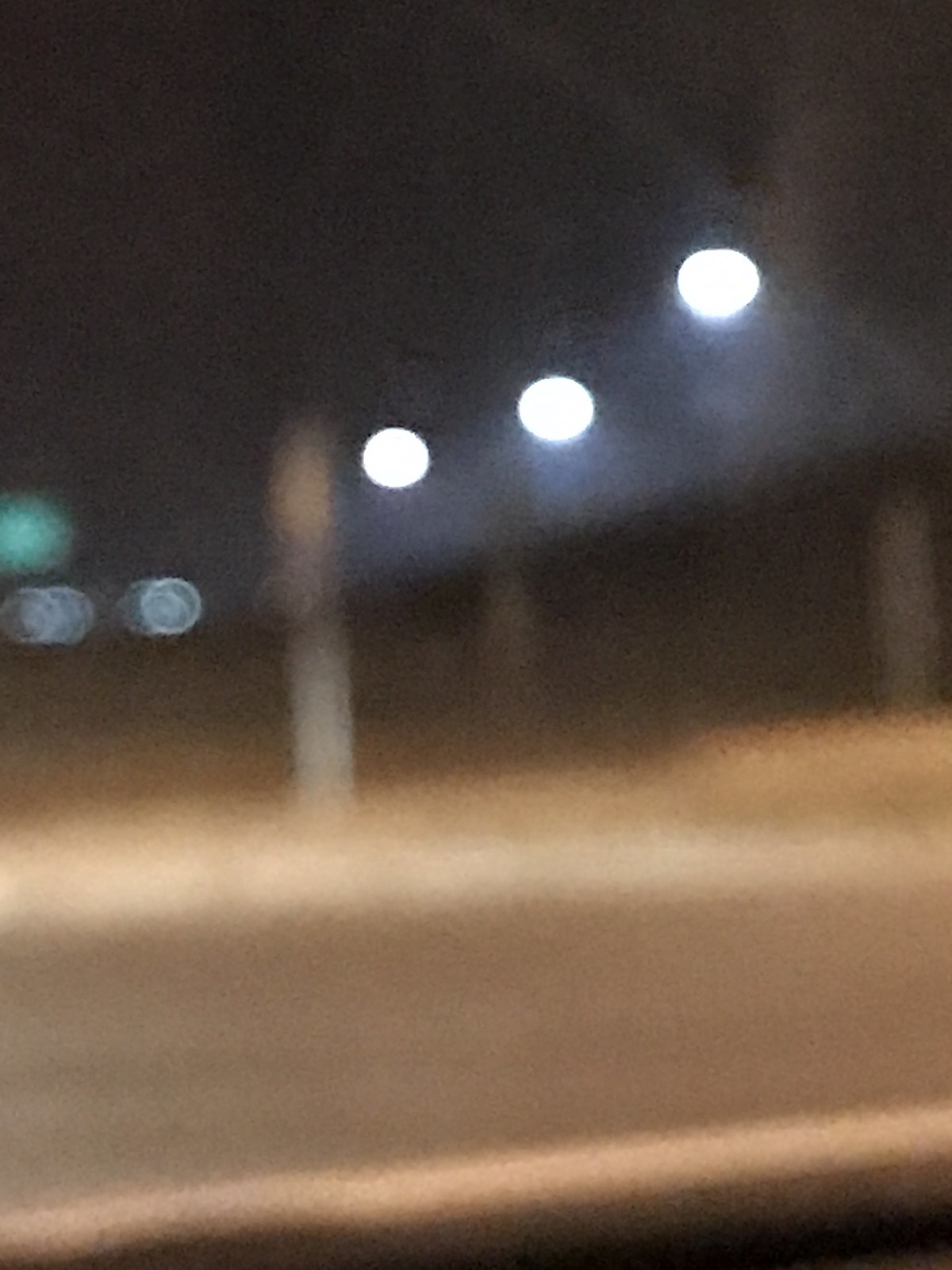The image is an outdoor, color photograph taken at nighttime and is extremely blurry and grainy. In the foreground, there is a dark tan street that curves horizontally across the mid-center of the image with a light-colored curb. To the left of center, a faint street sign or pole is visible on the sidewalk, though its details are indiscernible due to the blur. Toward the upper half of the image, three bright white spots—likely street lamps—form a loose diagonal pattern. One light is left of center, one is right of center and slightly higher, and the third is further to the right and higher still. These lights emit a bell-shaped pattern of illumination. The upper portion of the image transitions to pitch-black darkness. On the left edge, midway up, there is a faint green light possibly indicating an illuminated traffic or highway sign. There are no cars, people, or visible text in the photograph.